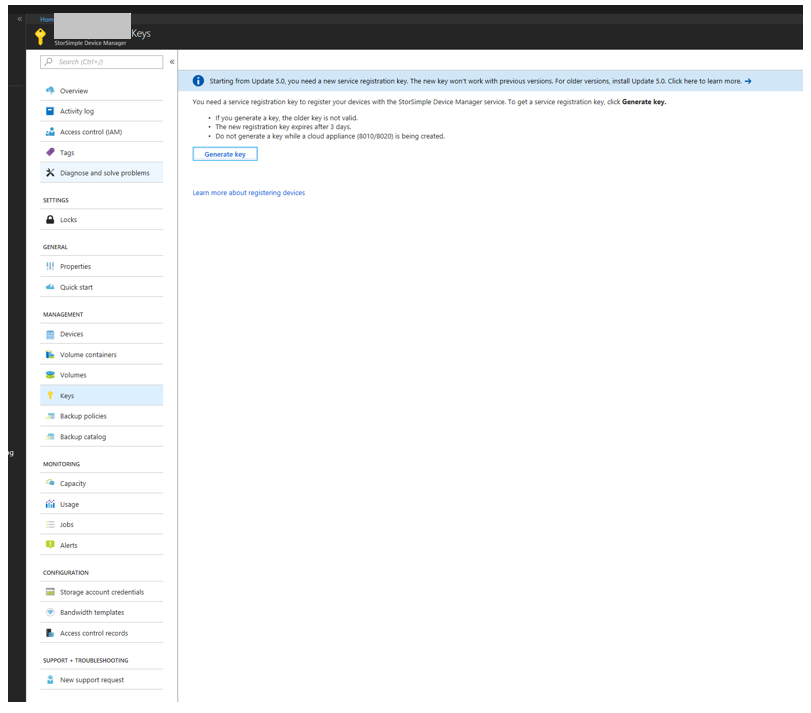In the image, there is a left-hand sidebar menu featuring multiple categories listed vertically. Each category has a corresponding icon and contains various sub-sections. From top to bottom, the categories and their details are as follows:

1. **Overview**
   - **Activity Log**
   - **Access Control**
   - **Tags** (accompanied by a shopping tag icon)
   - **Diagnose and Solve Problems** (with a wrench icon)

2. **Settings** (displayed in a gray color)
   - **Locks** (alongside a lock icon)

3. **General** (also in gray)
   - **Properties**
   - **Quick Test**

4. **Management**
   - **Devices**
   - **Volume Containers**
   - **Volumes**
   - **Cases**
   - **Backup Policies**
   - **Backup Catalog**

5. **Monitoring**
   - **Capacity**
   - **Usage**
   - **Jobs**
   - **Alerts**

6. **Configuration**
   - **Storage Account Credentials**
   - **Bandwidth Templates**
   - **Access Control Records**

Each section is distinctly organized with specific sub-sections, making navigation through various functionalities clear despite the slight blurriness of the image.